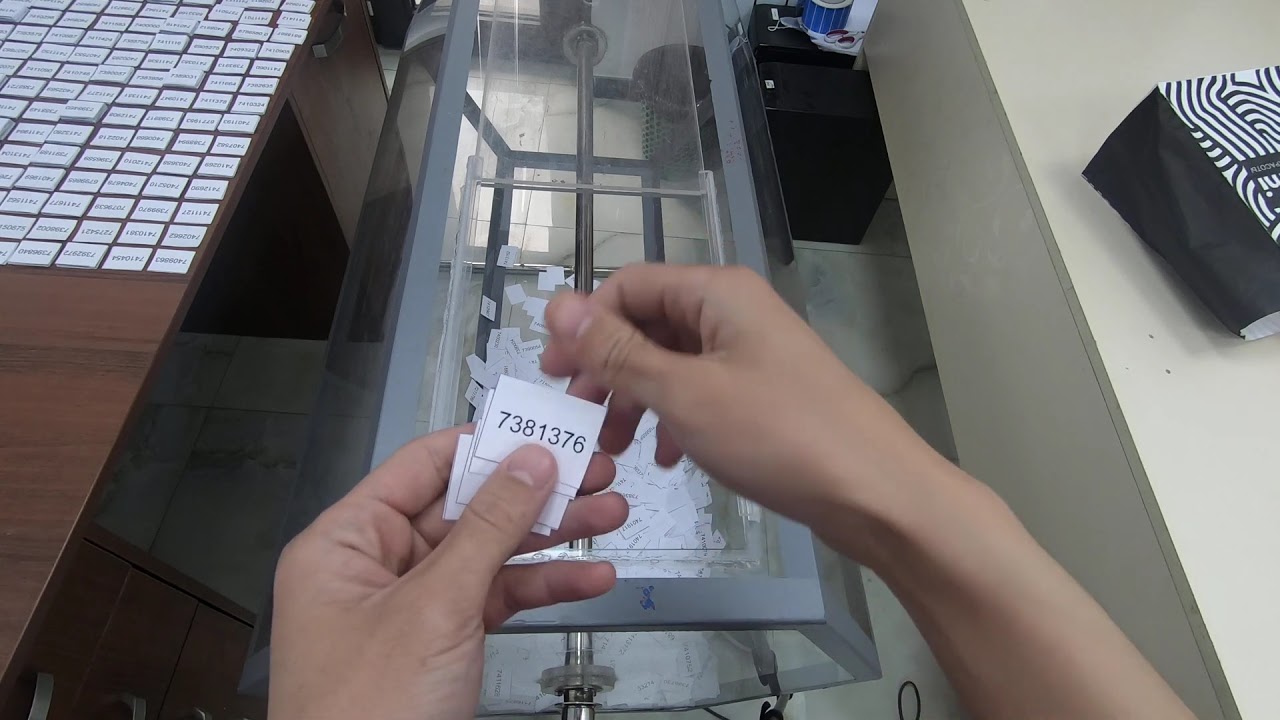In the foreground of this image, a person’s hands are visible, holding multiple small white slips of paper with black numbers 7381376 printed prominently. The individual appears to be in the process of placing or perhaps throwing these slips into a long, narrow acrylic plastic container with gray edges that already contains several similar pieces of paper. On the left side of the image, there is a brown wooden desk with three drawers at the bottom, neatly stacked with rows of more numbered slips. To the right, a white desk is visible, featuring a distinctive black-and-white paper bag with black sides. The setting suggests a scene related to organizing or perhaps a raffle event, with the mechanical drum-like container being used to collect the numbered slips.